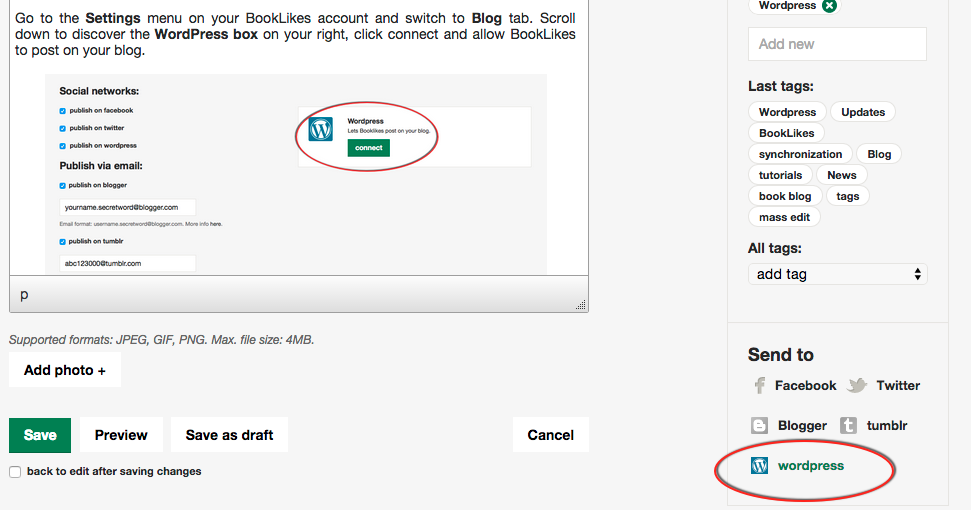The image displays a WordPress settings web page featuring various sections and options. On the far right side, there is a column labeled "WordPress" accompanied by an 'X' icon. Directly below this, a white rectangular box with the "Add New" option is visible. Further down, black text reads "Tags:" followed by various buttons labeled as WordPress, Updates, Book Likes, Synchronization, Blog, Tutorials, News, Book Blog, Tags, Mass Edit, and All Tags. Additionally, there's an option to add a tag.

Next, there's a feature for sharing content to different social media platforms: Facebook, Twitter, Blogger, Tumblr, and WordPress. To the left side of the image, there’s a visual guide showing the steps to integrate a Book Likes account with a WordPress blog. It instructs users to navigate to the settings menu on their Book Likes account, switch to the blog tab, and scroll down to find the WordPress box on the right. Users are then prompted to click "Connect," allowing Book Likes to post on their blog. This guide includes images of the WordPress logo and a circular "Connect" button.

Below these instructions, multiple buttons are displayed: a green "Save" button, a "Preview" button, a "Save and Stop" button, and a "Cancel" button.

In summary, the image is a detailed instructional screenshot from a WordPress settings page, offering options for managing tags, social media synchronization, and providing a step-by-step guide for connecting a Book Likes account to a WordPress blog, with clear call-to-action buttons at the bottom for saving or canceling changes.